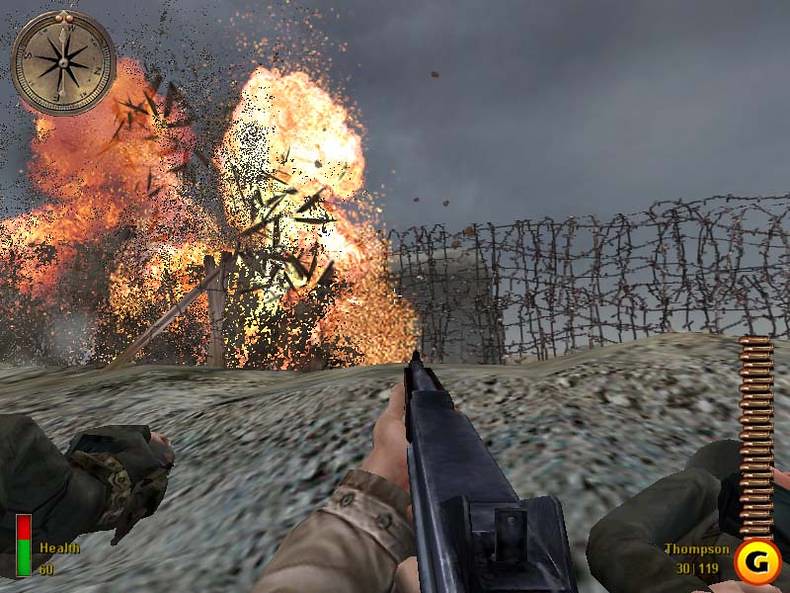This screenshot captures an intense moment from a first-person shooter video game, offering a highly immersive protagonist's perspective. At the center of the image, a modern assault rifle is prominently featured, with its barrel extending towards the middle of the screen. The protagonist's left hand is gripping the weapon firmly. 

To the left side of the image, a dramatic explosion is in full force, sending flames and splintering wood in all directions, adding to the chaos and urgency of the scene. Nearby, barbed wire is visible, suggesting that the area is heavily fortified or within a warzone.

In the upper left corner, a brass compass indicates a western direction, crucial for navigation. In the lower left corner, another character’s hand can be seen, hinting at a cooperative or multiplayer scenario. Below, a health meter displays the current health status at 60, represented with a red top and green bottom.

On the far right side, a vertical column shows the remaining ammunition, and directly beneath it, the letter “G” is visible, potentially denoting a keybinding or game control.

Overall, this image encapsulates the high stakes and action-packed nature of the game environment.